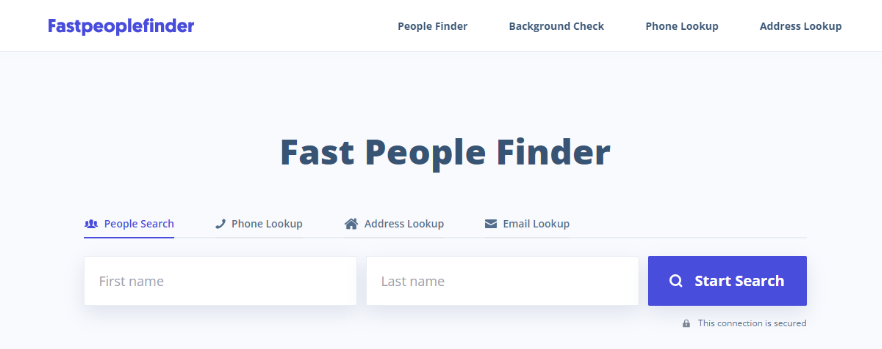The image depicts the homepage of the website "Fast People Finder." In the upper left-hand corner, the website's name is prominently displayed in purple text against a horizontally stretched net-like background. Below this, a menu bar is visible with options such as "People Finder," "Background Check," "Phone Lookup," and "Address Lookup," all written in gray.

Beneath the menu bar, there's a light blue box prominently featuring the website's name, "Fast People Finder," in large dark gray letters. Within this box, "People Search" stands out in purple text with a purple underline, indicating it as the selected option. Positioned next to "People Search" are the additional capabilities "Phone Lookup," "Address Lookup," and "Email Lookup."

Central to the page, two adjacent white search bars invite users to input their first and last names, respectively. To the right of these search fields, a smaller purple box features a search icon along with the phrase "Start Search" in white text. At the bottom of the page, a fine print message assures users that "This connection is secured," accompanied by an icon of a black lock.